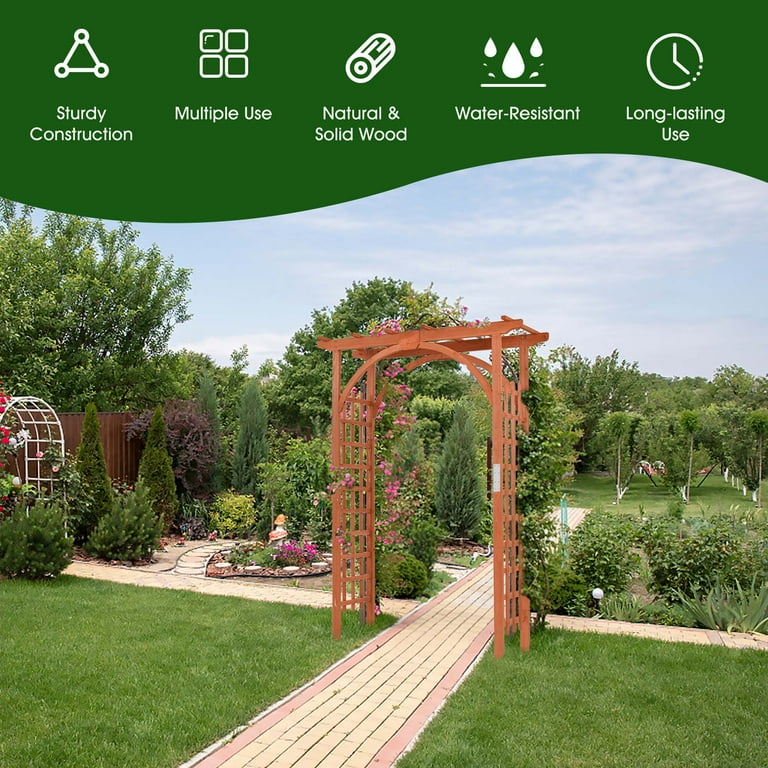This photograph captures a meticulously landscaped garden that could be the setting for a beautiful backyard wedding. In the foreground, a T-shaped brick walkway paved with tan bricks outlined in red starts slightly left of the center and extends diagonally downward, dividing the lush green grass on either side. Midway along the path, a charming light brown wooden trellis adorned with climbing flowers forms an inviting small archway. To the left of this trellis, a small rock garden emerges, flaunting vibrant pink flowers.

Further beyond, another horizontal brick path intersects the first, creating the T-shape. Adjacent to this intersection on the left, a variety of shrubs, flowers, and plants including clusters of yellow and purple flowers, embellish the garden, while a tall brown fence provides a backdrop. On the right, orderly rows of plants and an expanse of grassy terrain stretch out toward the back.

A white archway covered in delicate white and pink flowers can be seen near the left-hand side against the brown fence. In the distance, lines of trees complete the scenic vista under a light blue sky with wispy clouds. Notably, adding a commercial touch, labels indicating 'sturdy construction,' 'multiple use,' 'natural and solid wood,' 'water-resistant,' and 'long-lasting use,' are subtly overlaid at the top, set against a wavy green banner, possibly hinting at this image being part of an advertisement.